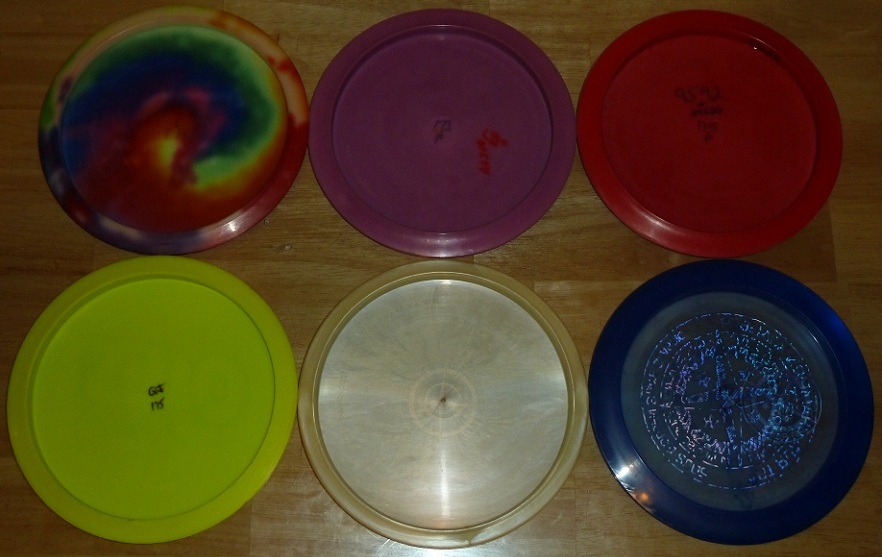This photograph features six round plastic lids for containers, arranged in two rows of three, set against a light laminate wood floor. Despite the dim lighting, the vibrant colors of each lid stand out. In the top row from left to right, the first lid showcases a tie-dye pattern with rainbow hues, while the second lid is purple adorned with black and red markings. The third lid in this row is red, also featuring some black writing. On the bottom row, starting from the left, the first lid is chartreuse green with black writing in the center, followed by a light golden-colored lid. The final lid on the bottom right is dark blue with a lighter blue four-pointed star design in the center, all resting closely together in a tidy arrangement.